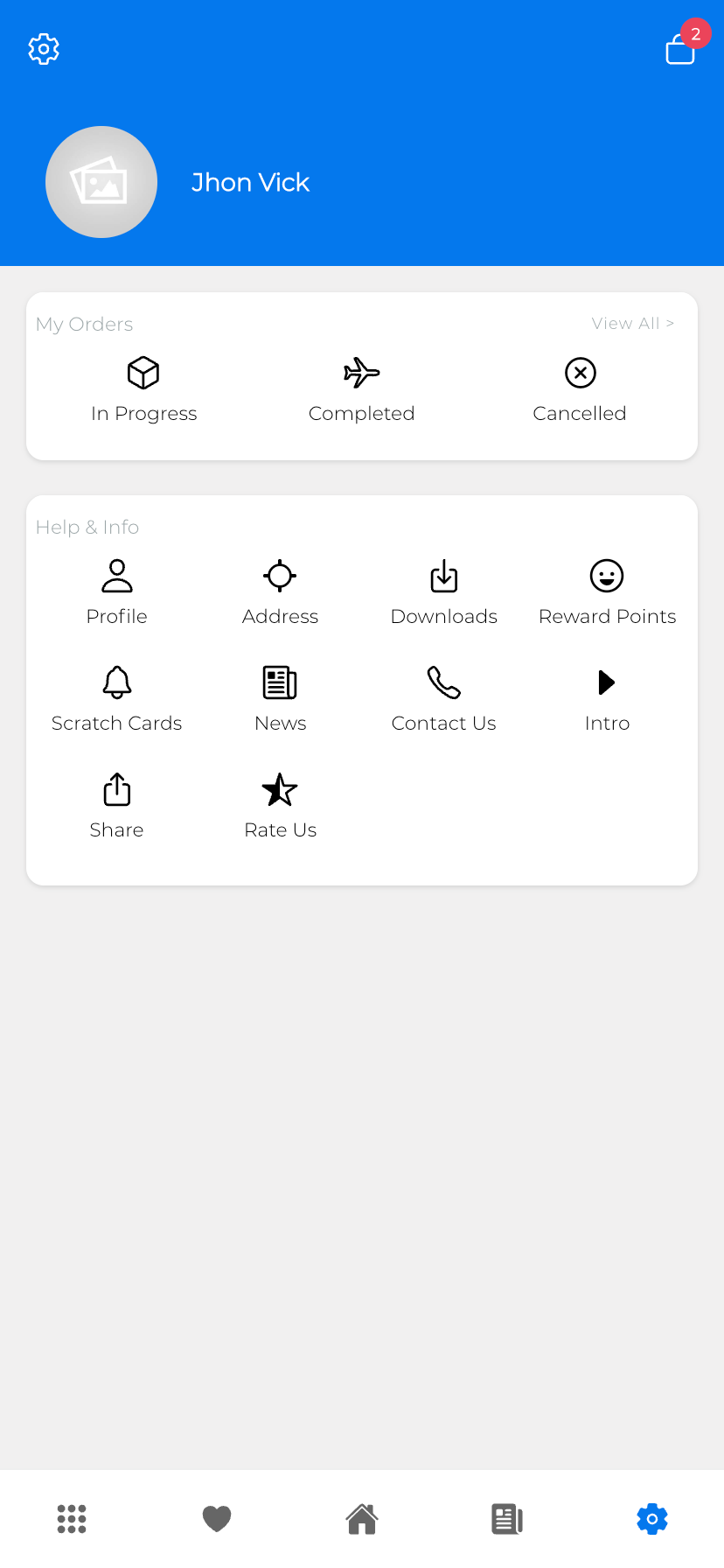This is a detailed mobile phone screenshot, likely from an Android or Google device, displaying an unknown application interface. The screenshot features a blue banner at the top-left corner with a round, empty icon and the name "JohnVic" (spelled J-O-N-V-I-C-K).

Below the banner, there are two primary sections:

1. **My Orders Section**: 
   - Comprises three labeled options: In Progress, Completed, and Canceled.
   - A "View All" button is located in the upper right-hand corner of this segment.

2. **Help & Info Section**:
   - Contains ten icons labeled: Profile, Address, Downloads, Reward Points, Scratch Cards, News, Contact Us, Intro, Share, and Rate Us.

The bottom half of the screenshot appears empty, apart from these segments.

Additional interface elements include:
- A checkout button in the upper right-hand corner with a shopping bag icon indicating two items.
- A settings gear icon on the left-hand side.

The default bottom menu includes:
- An apps button,
- A favorites heart button,
- A home button,
- A news icon,
- A blue settings button.